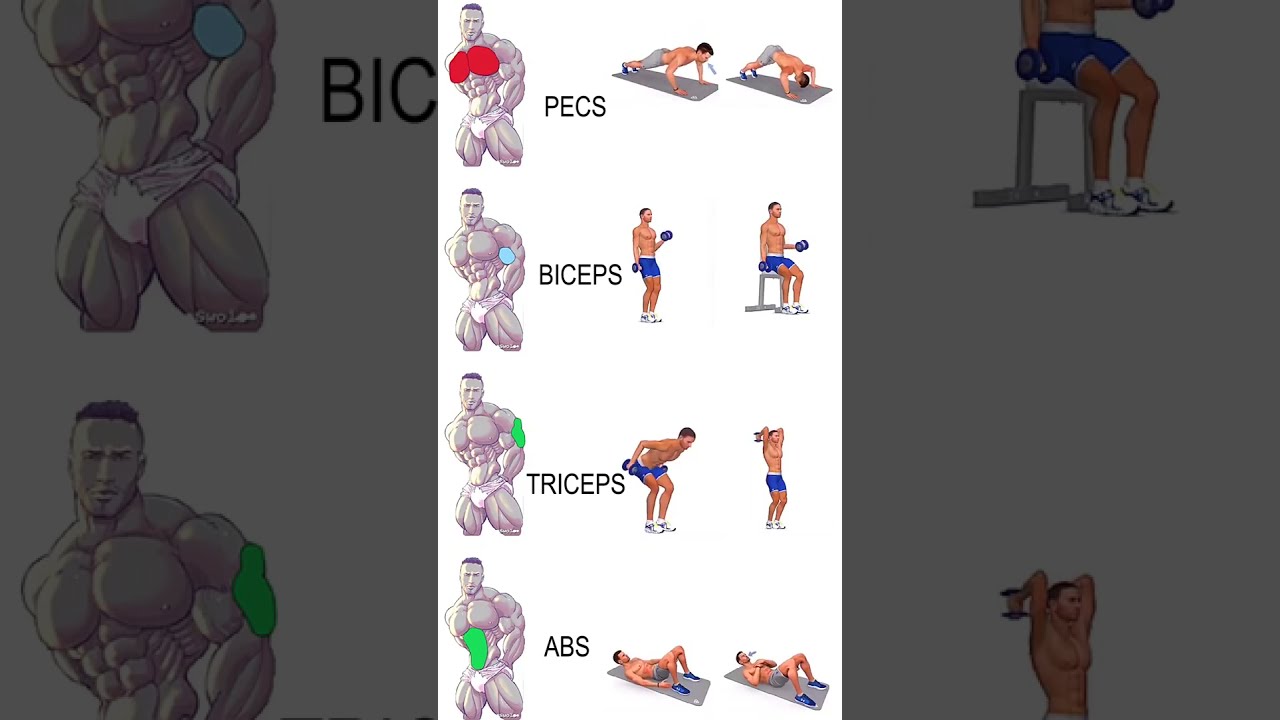The image is a detailed, educational chart showcasing various exercises targeting specific muscle groups, accompanied by illustrations. The chart is divided into three main sections: the left side features an illustrated bodybuilder, the center lists the names of the muscle groups, and the right side demonstrates corresponding exercises.

In the center, four rows detail exercises for the pecs, biceps, triceps, and abs. Each muscle group is paired with an illustration of the bodybuilder on the left, highlighting the targeted area in different colors—red for pecs, blue for biceps, green for triceps, and green again for abs.

1. **Pecs (chest) Exercises:** The top row highlights the pectoral muscles in red. Next to it, a sequence shows an individual performing various push-up variations, starting from a standard position to a stance where their butt is lifted.
   
2. **Biceps Exercises:** The second row highlights the biceps in blue. Adjacent to it, there are illustrations of a person doing standing dumbbell curls followed by seated dumbbell curls.

3. **Triceps Exercises:** In the third row, the triceps are highlighted in green. The illustrations show a person performing tricep kickbacks and overhead tricep extensions, raising their hands above their head from a standing position.
   
4. **Abs (abdominal) Exercises:** The bottom row focuses on the abdominal muscles, again highlighted in green. The corresponding workout illustration shows a person on a mat, performing crunches or half sit-ups with their knees bent.

This well-structured chart is a comprehensive guide for fitness enthusiasts, visually linking each muscle group with targeted exercises to develop a stronger physique.